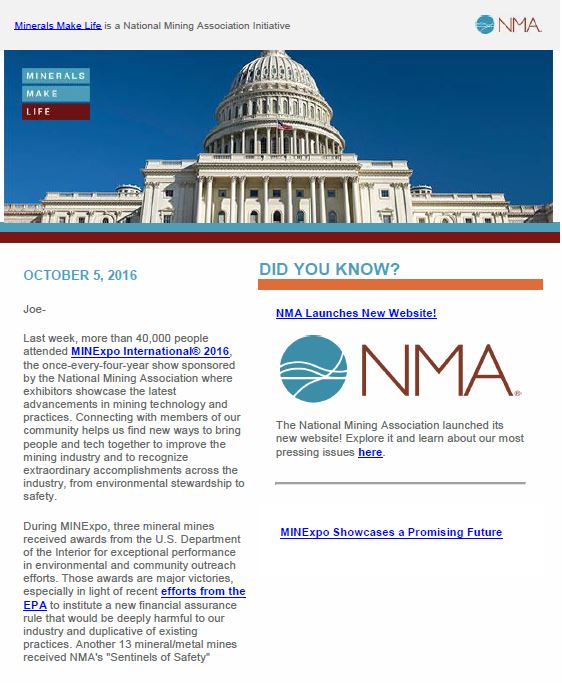**Website Category: Minerals Make Life - A National Mining Association Initiative**

**Image Description:**

In the top right corner of the image, there is a logo of the National Mining Association (NMA). The main visual element features a striking picture of a capitol building under a clear sky, symbolizing governance and regulation. 

**Caption:**

"Minerals Make Life - October 5th, 2016: Last week, more than 40,000 attendees gathered for MINExpo International 2016, a premier event hosted every four years by the National Mining Association (NMA). Exhibitors at the expo presented cutting-edge mining technologies and practices. This event fosters connections within the mining community, driving innovation and collaboration to advance the industry. During MINExpo, three exceptional mineral mines were honored by the U.S. Department of the Interior for their achievements in environmental management and community engagement. These accolades mark significant triumphs, particularly amidst ongoing challenges posed by potential new EPA regulations that could adversely affect the industry."